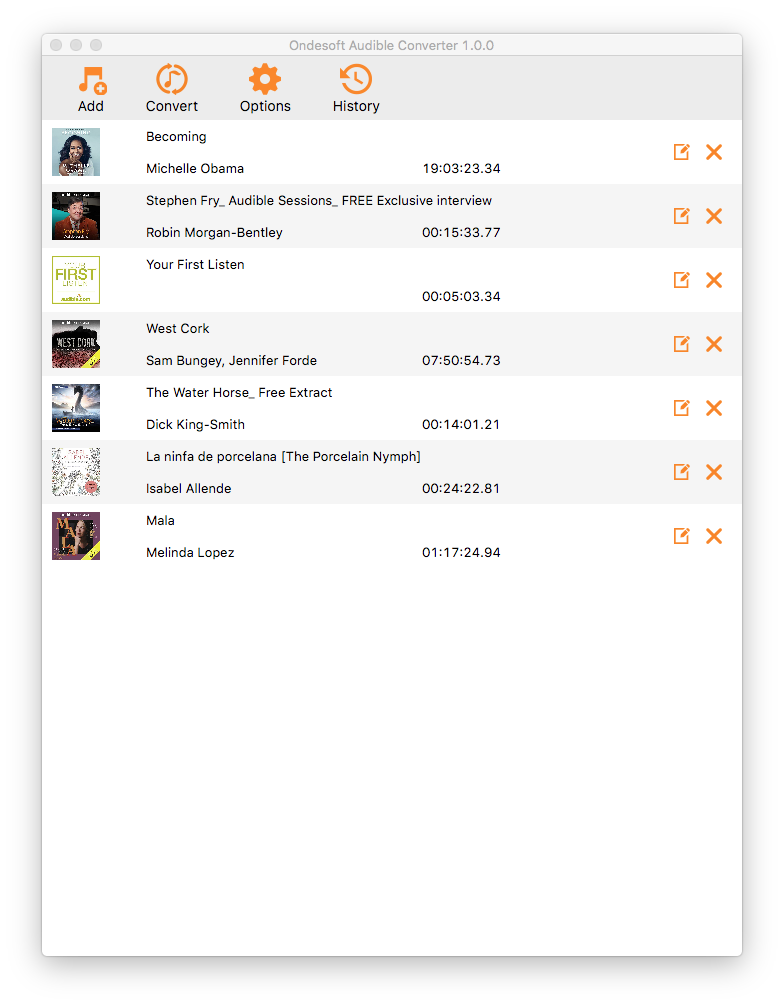The screenshot displays the interface of the Ondesoft Audible Converter 1.0.0 software running on a Mac OS. The main window shows a list of audiobooks presumably sourced from the Audible platform. Among the titles visible are "Becoming" by Michelle Obama and another work by Stephen Fry. There's also a generic entry titled "Your First Listen" along with additional unidentified audiobooks.
 
Each audiobook listing includes information that appears to be the total length of the audiobook, with some durations displaying unusually long times, like 19 days for "Becoming" by Michelle Obama, which may indicate a misinterpretation or error. The interface features buttons and options such as "Add," "Convert," and "History," suggesting the software's purpose is to convert audiobooks to different file formats, potentially for easier access or compatibility.